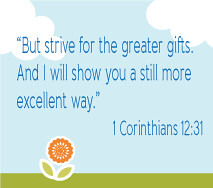The image is designed like a simple yet artistic poster, featuring a light blue background that depicts a cartoon sky with two white clouds—one in the top left corner and the other in the top right. In the center, a Bible quote in dark blue text reads: "But strive for the greater gifts, and I will show you a still more excellent way. 1 Corinthians 12:31." At the bottom of the image, a horizontal olive green stripe represents grass, accentuated by a small, circular flower with orange and yellow petals and two green leaves at its base. The overall composition effectively uses clean, minimalistic elements to convey a message of inspiration and hope.